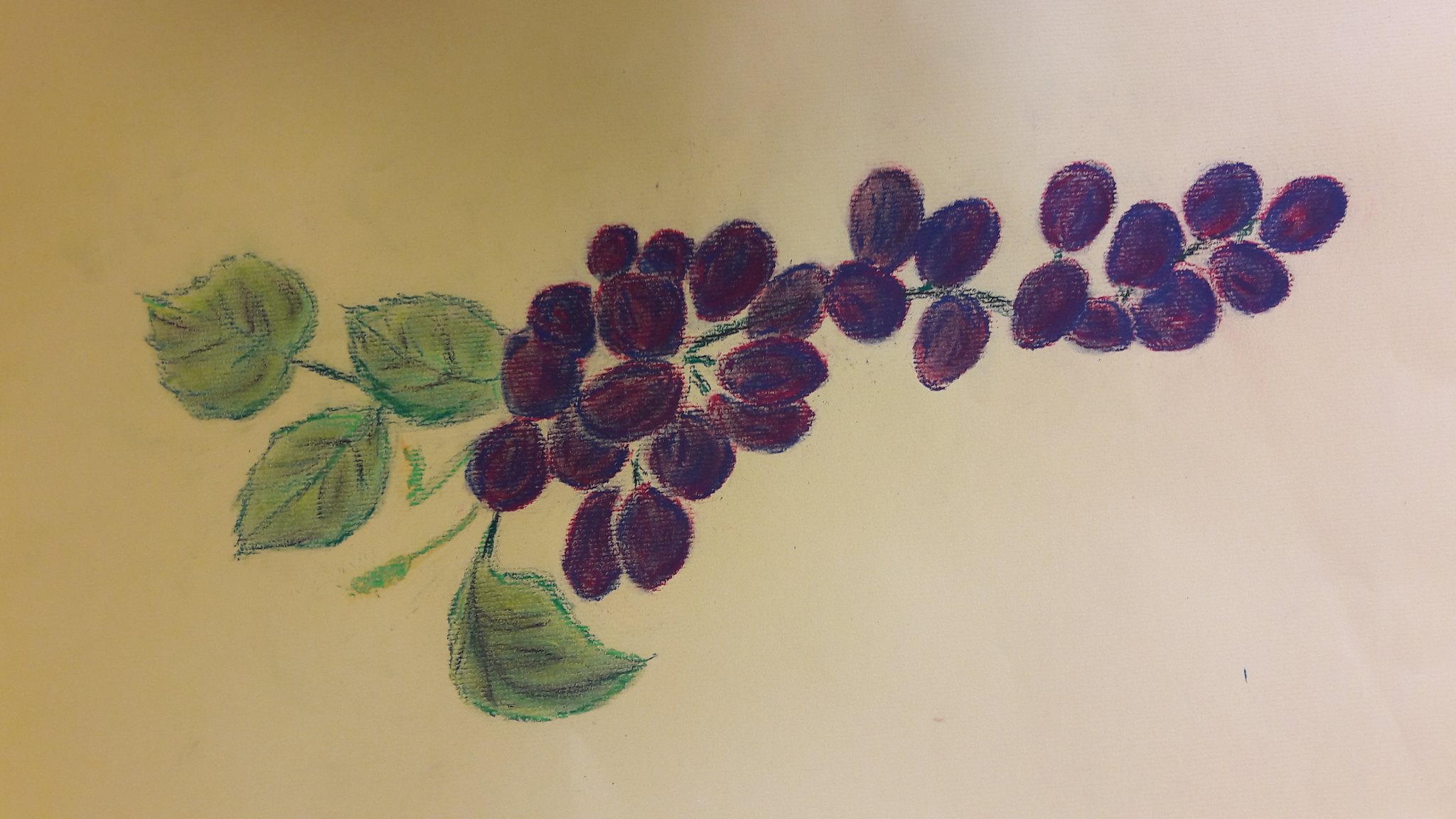The image is a wide, color illustration on a piece of paper with two tones: a lighter cream beige on the right, transitioning to a more yellow tone towards the left. This landscape-oriented artwork features a detailed bunch of red grapes attached to a vine. The grapes, numbering about 20, display a rich wine or maroon color with streaks of lighter and darker hues, giving them a three-dimensional appearance. Interspersed among the grapes, the green vine can be partially seen, while in other areas it is obscured by the arrangement of the fruit.

On the left side of the illustration are four intricately detailed green leaves. These leaves extend in various directions and show intricate lines and shading, with darker green accents around the edges and touches of black to define their veining. The artwork resembles an oil painting due to its texture and subtle reflections, suggesting it is not created with pencils or felt-tip markers. The background transitions from a very light pink on the right to a golden color on the left, adding depth to the scene. There are no people, animals, flowers, buildings, or signs in the image, which solely focuses on the natural beauty of the grapevine.